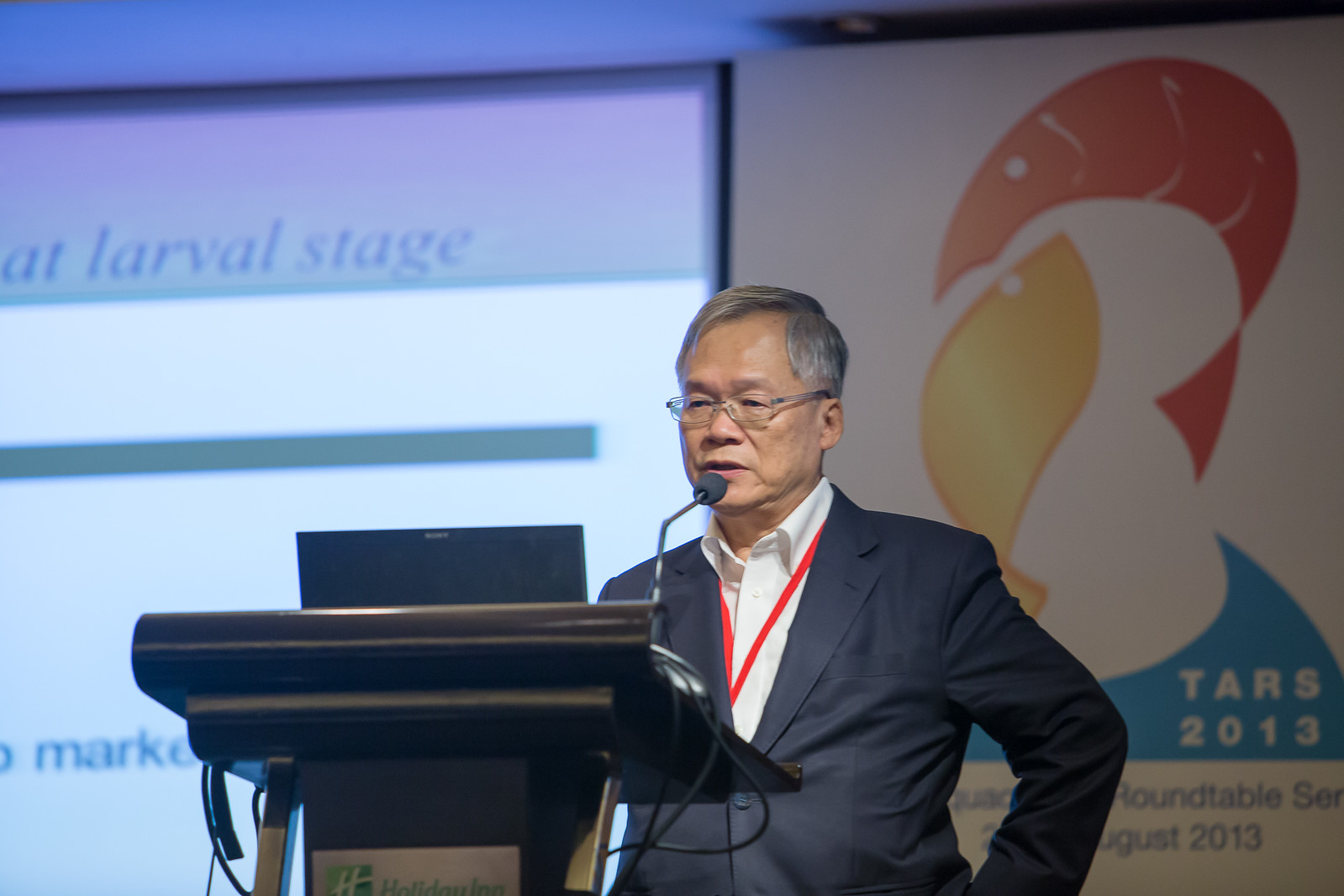This detailed photograph captures an older Asian man with short, parted gray hair and smooth skin, indicating his age primarily through his graying hair. He is standing at a black podium adorned with cords and an open laptop, speaking into a black-tipped microphone. He wears sleek, thin rectangular glasses, a dark blue business jacket, a white button-down shirt, and a red lanyard around his neck, suggestive of his participation in a professional conference. Behind him, a large, brightly-lit screen displays part of a PowerPoint presentation featuring the words "larval stage" and "market," along with event signage that reads "TARS 2013" and "Roundtable 2013," accompanied by a red and yellow fish logo. The setting, which appears to be at a Holiday Inn based on the podium's branding, suggests that he may be presenting scientific research.